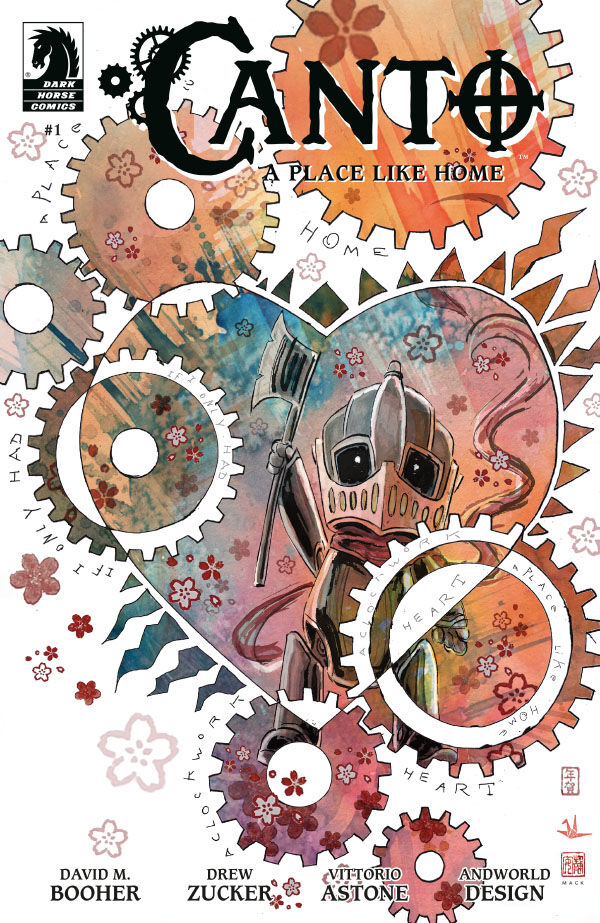The image is a semi-abstract watercolor painting serving as a comic book cover for Dark Horse Comics. Prominently featured in the upper left corner is the Dark Horse Comics logo, a small white square housing a black horse. A wooden, knight-like figure, adorned in armor and wielding an axe, stands at the core of the composition. This knight's face is shielded by what appears to be a metal mask with two white eye slits. Surrounding the figure are a plethora of gears that span from top to bottom, in varying shades of pinks, oranges, and occasionally blues and purples, often adorned with floral patterns. In the heart of the cover—literally, a pink and blue-purple heart scattered with flowers—resides this armored figure. The gears display words like "Heart," "Clockwork," "If I Only Had," and "Home," suggesting a whimsical, yet intricate, theme that merges mechanical elements with themes of emotion and identity.